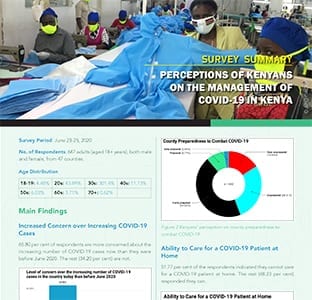This low-quality image appears to have been sourced from a website or a PDF document. It features a text-based dashboard layout with infographics and data. At the top of the image, there is a photograph set in a factory environment where workers are seated at sewing machines, manufacturing blue overalls for medical use. The workers are wearing masks. 

Overlaying the image is text that reads, "Survey Summary: Perceptions of Kenyans on the Management of COVID-19 in Kenya." Below the photo, a light green background hosts two columns detailing the survey period and main findings. Though the text is largely blurry and difficult to read, there is a partially visible bar graph in the top section and a pie chart further down, providing visual representation of some key data points.